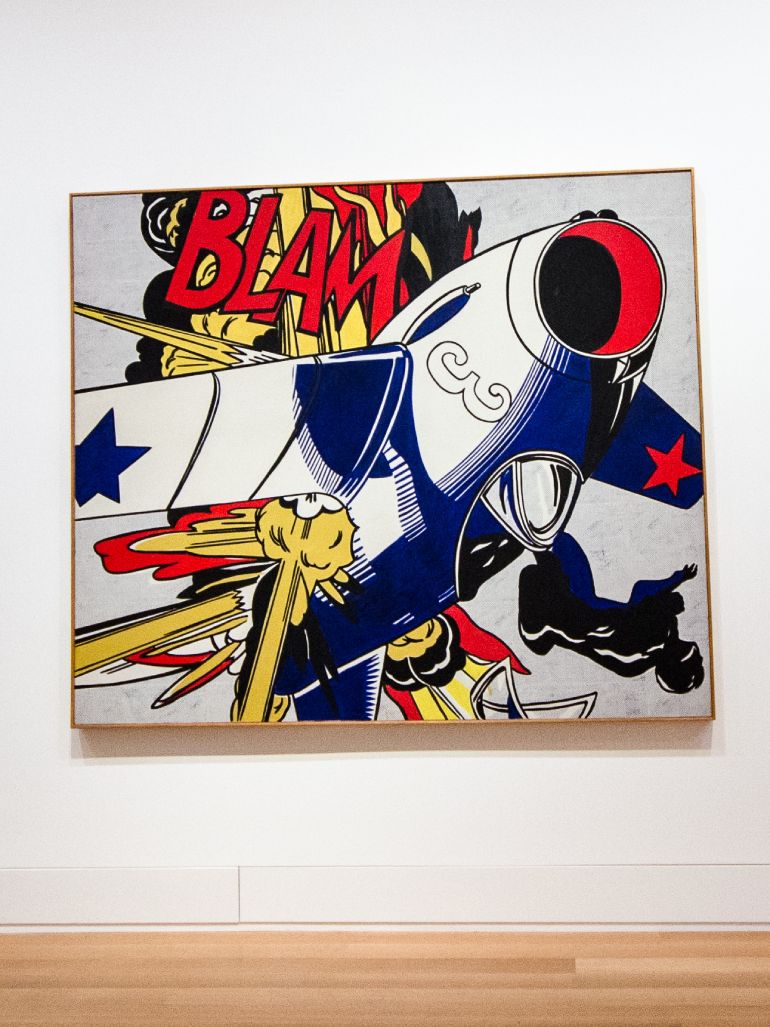This vertical rectangular artwork features a vivid, animated depiction of a chaotic mid-air scene. Dominated by a colorful, upside-down airplane marked with the number three, the piece showcases a dramatic moment frozen in time. The aircraft, primarily black, blue, and white, displays a distinguishing blue star on one wing and a red star on the other. An open, black and red cockpit reveals a pilot figure seemingly ejected from the seat, spiraling towards the image's bottom right. The air around this scene feels charged with energy, accentuated by an explosive "BLAM" written in bold red letters against a burst of red, yellow, and black. Additional fragments of this explosion are visible near the plane’s wing, suggesting an impactful collision. The backdrop of the scene is a grayish-white, sitting above a light brown wood panel that appears to be part of a frame but is cut off. The artistic nature of this piece, reminiscent of Dr. Seuss's whimsical style, makes it evident that it’s not a photograph but a crafted graphic artwork displayed on a white wall above a wooden floor.